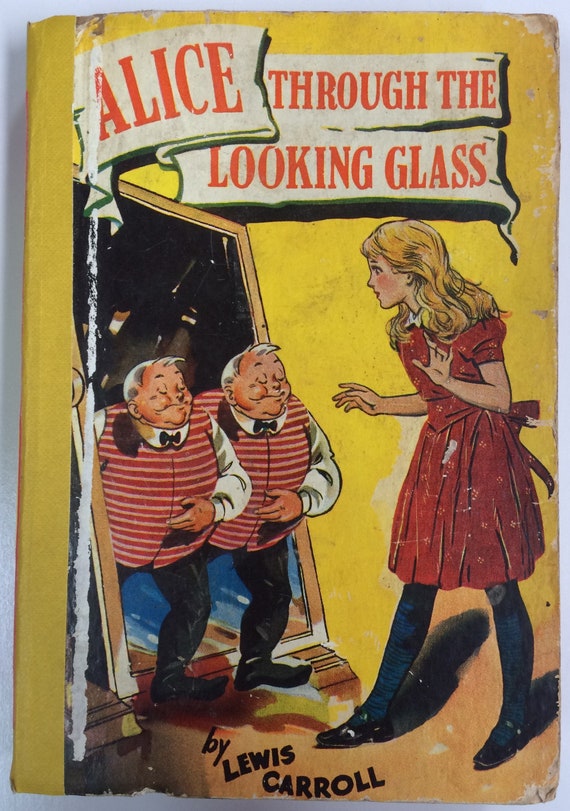The book cover for "Alice Through the Looking Glass" by Lewis Carroll features a vibrant yellow background that gradients into a peach color near the bottom right. Dominating the right side of the cover is an illustration of Alice, depicted with long, wavy blonde hair cascading over her shoulders. She is dressed in a red dress tied in a bow at the back, dark tights, and black shoes. Alice stands with her hands raised, appearing startled as she gazes at two shorter, older men emerging from a doorway. These men, identically dressed in waiter-like outfits with red and white striped vests, white shirts, black bow ties, black pants, and black shoes, have gray hair and eyes closed in seemingly cheerful expressions. At the top of the cover, the title "Alice Through the Looking Glass" is displayed in red text on a white banner, while the author’s name, "By Lewis Carroll," is printed in black text at the bottom center. The illustration style is vintage, evoking a classic print publication aesthetic.